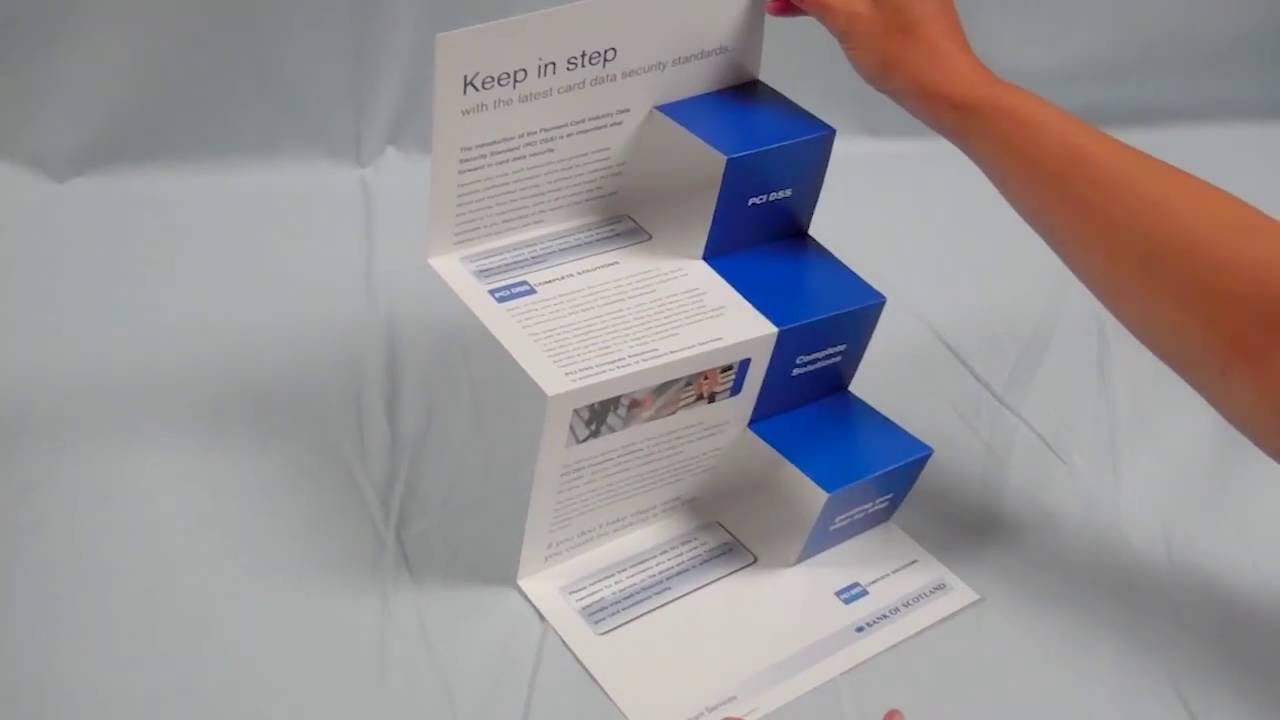The image is a rectangular, close-up shot of a brochure held against a white, crinkly fabric background, possibly a bed sheet. An arm with a pinkish tan complexion, visible from the elbow down, is reaching in from the right edge of the picture, with fingers grasping the side of the brochure. The brochure itself is unfolded and resembles a small staircase thanks to its accordion-style creases. The ad measures about 8.5 by 14 inches and features four rectangular sections. At the top, in large blue sans-serif font, it reads "Keep in step," followed by the phrase "with the latest card data security standards." The right side of the brochure displays blue steps, reinforcing the staircase look. At the bottom, the Bank of Scotland logo is visible. While the brochure contains a lot of text, it is too fine to be clearly read in the image.